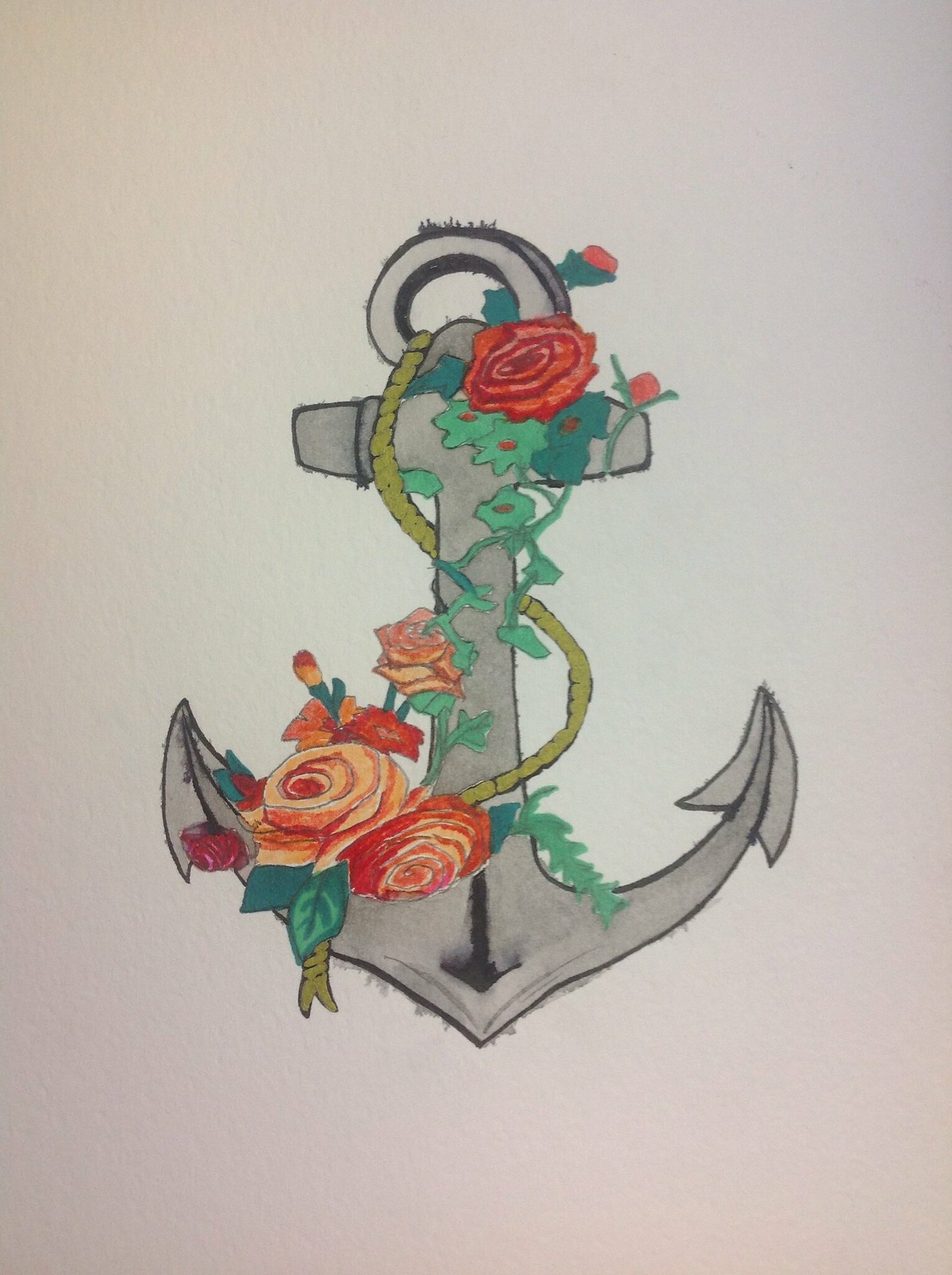This stunning illustration features a grayish-silver anchor intricately adorned with vibrant floral patterns. Red roses, green leaves, and other delicate flowers entwine the anchor, giving it a lively and organic feel. A yellowish rope snakes through the floral elements and the anchor itself, adding a dynamic sense of movement reminiscent of a vine. The detailed and vivid artwork is set against a pristine white background, emphasizing the colors and textures of the anchor and its adornments. This piece, with its intricate design and bold use of color, could easily be envisioned as a tattoo or a standalone piece of art.